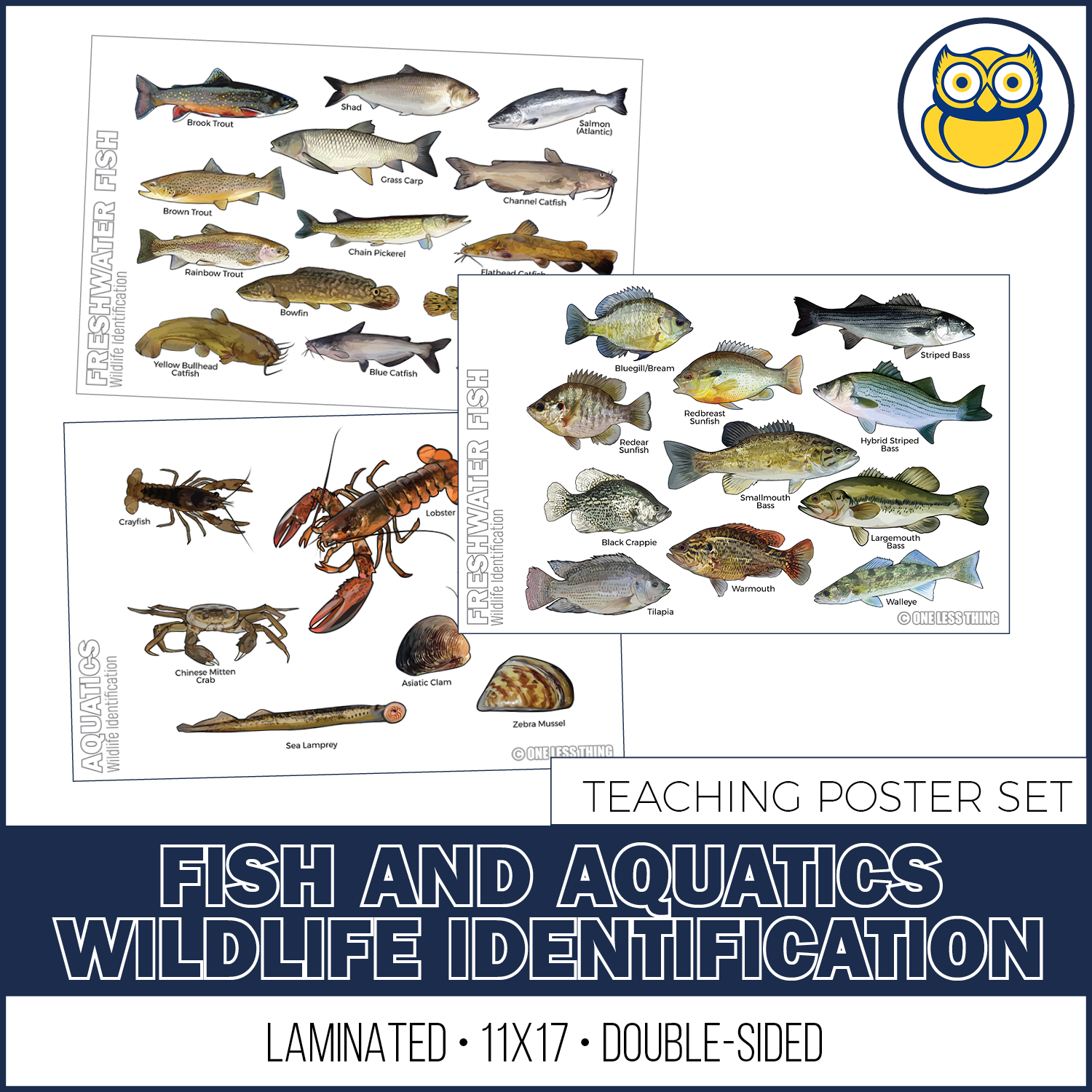This image features a detailed teaching poster set for Fish and Aquatic Wildlife Identification. In the upper right-hand corner, there is a gold and blue owl icon enclosed in a black circle, representing the publisher, One Less Thing. The main header, "Fish and Aquatic Wildlife Identification," is prominently displayed in bold, white text against a blue border. The entire set is advertised as laminated, 11 by 17 inches, and double-sided, with "Teaching Poster Set" written at the bottom in black text.

The image showcases three individual identification cards. The first two cards are labeled "Freshwater Fish Wildlife Identification" and display a variety of traditional freshwater fish species, including trout, shad, salmon, carp, pickerel, various types of catfish, bream, sunfish, bass, crappie, tilapia, walleye, and striped bass. Each fish is depicted in full color with its name printed beneath.

The third card, labeled "Aquatics Wildlife Identification," highlights aquatic creatures such as crayfish, lobsters, clams, mussels, lampreys, and Chinese mitten crabs. These colorful illustrations provide clear, detailed visuals of each species, making it easy for viewers to identify them. The meticulous artwork and organization of these cards offer both educational value and aesthetic appeal.